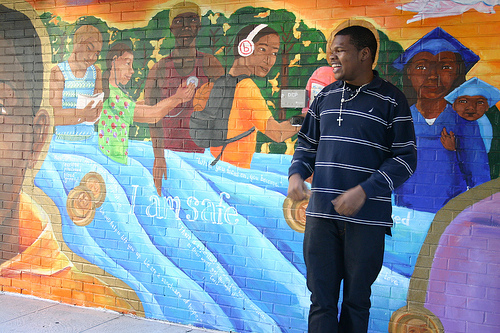In this vibrant outdoor, daytime photograph, an African-American man stands smiling in front of a detailed and colorful mural on a brick wall. He is wearing a long-sleeved navy blue shirt with white horizontal stripes, black pants, and a gold cross necklace. His short dark hair complements his bright demeanor as he looks slightly away from the camera.

The mural behind him features a rich tapestry of African-American figures engaging in various acts of kindness and learning, suggesting themes of community and safety. On the left, a head-and-shoulders portrait of a black man is depicted. Above him, a black individual, possibly a woman, wears a blue tank top and looks down at some paperwork. Next to her, a brown woman in a red and green shirt uses a stethoscope on a black man in a red shirt. Further to the right, a brown man with a black knapsack and pink and white headphones holds out his hand as if reaching for something. Another significant figure in the mural is a black man in a blue graduation cap and gown, standing beside a younger black person dressed similarly in a light blue cap and gown. The mural also features dynamic elements like ocean waves and prominently displays the phrase "I am safe" in white on its center. In the bottom right corner of the mural, there is a close-up of a purple head and shoulders, adding to the vivid and expressive nature of the artwork. The overall mural is imbued with hues of orange, blue, and purple, contributing to its vibrant aesthetic.